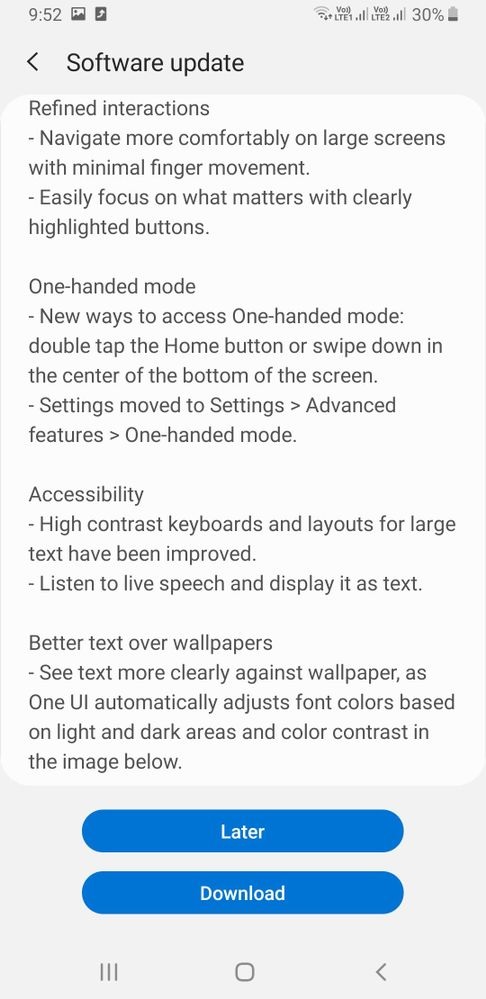This image is a detailed screenshot from a smartphone interface showcasing a software update notification. The top header features a very light gray background. On the left side of the header, the time is displayed in a gray font as "9:52", while the right side houses several icons: a battery icon indicating a 30% charge, wireless connection status, and a Wi-Fi connection indicator. Just below the header, "Software Update" is prominently written in bold gray font with a left-pointing arrow to its left.

The main body of the screenshot has a white background and is divided into several sections. The first line reads "Refined Interactions," followed by another section titled "One-Handed Mode," each accompanied by brief explanations. Further down, there are sections labeled "Accessibility" and "Better Text Over Wallpapers."

At the very bottom of the screenshot, two blue rectangular buttons with rounded corners are aligned vertically. The top button, labeled "Later," uses white font, while the bottom button reads "Download" in the same white font.